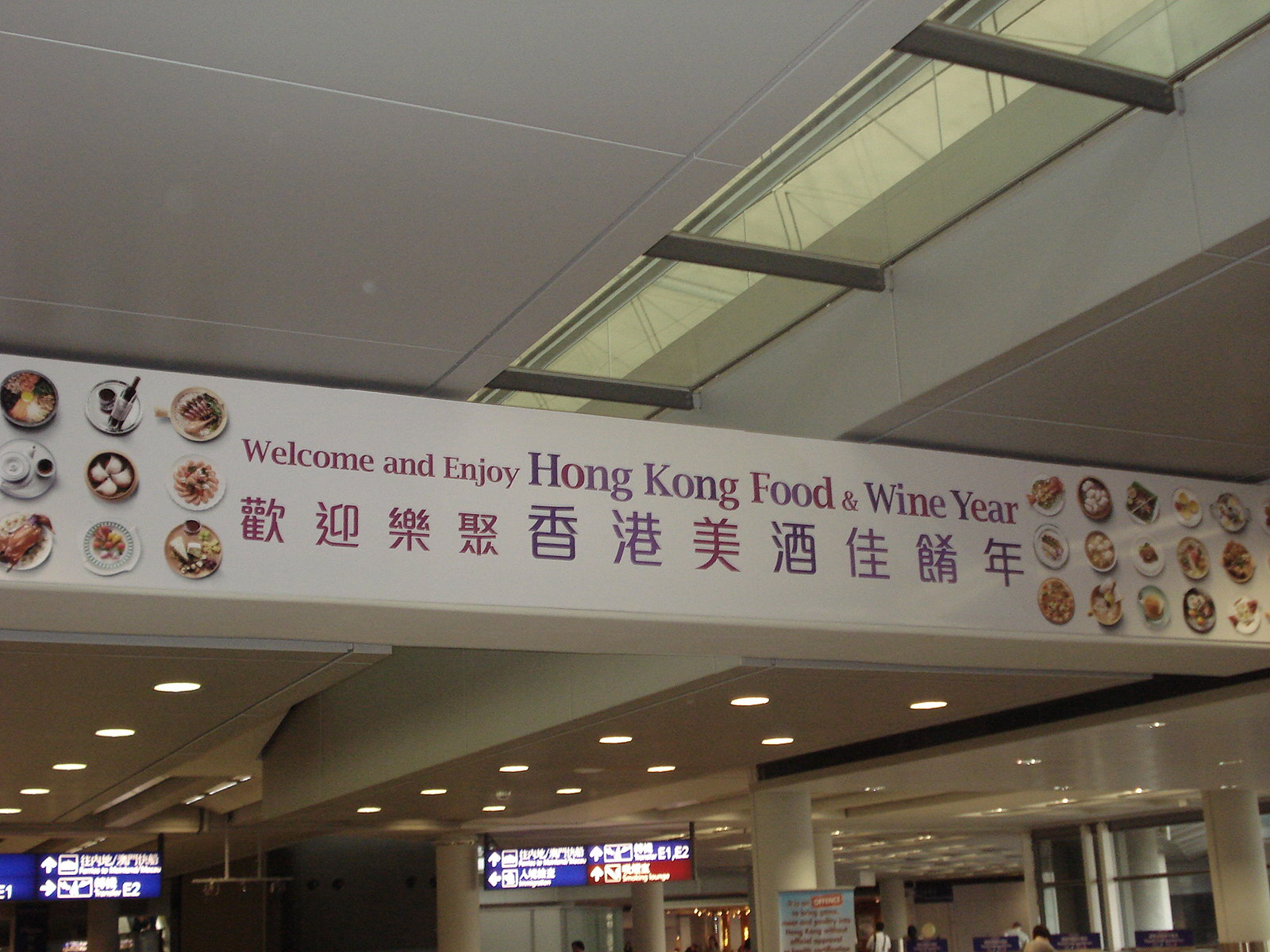The photograph captures a bustling transit terminal, likely an airport or train station in Hong Kong, adorned with a prominent welcoming banner. The top third of the image reveals the structural details of the ceiling, mostly gray and functional. Spanning the middle section, a long banner stretches across a beam, showcasing diverse Asian cuisines in vivid images on either end. The banner features text in both English and Chinese that reads, "Welcome and Enjoy Hong Kong Food and Wine Year," celebrating the city's rich culinary scene. The lower third of the image provides glimpses of the terminal below, filled with people and illuminated directional signs, guiding travelers to various destinations. The scene exudes a vibrant atmosphere, inviting visitors to explore the flavors of Hong Kong.